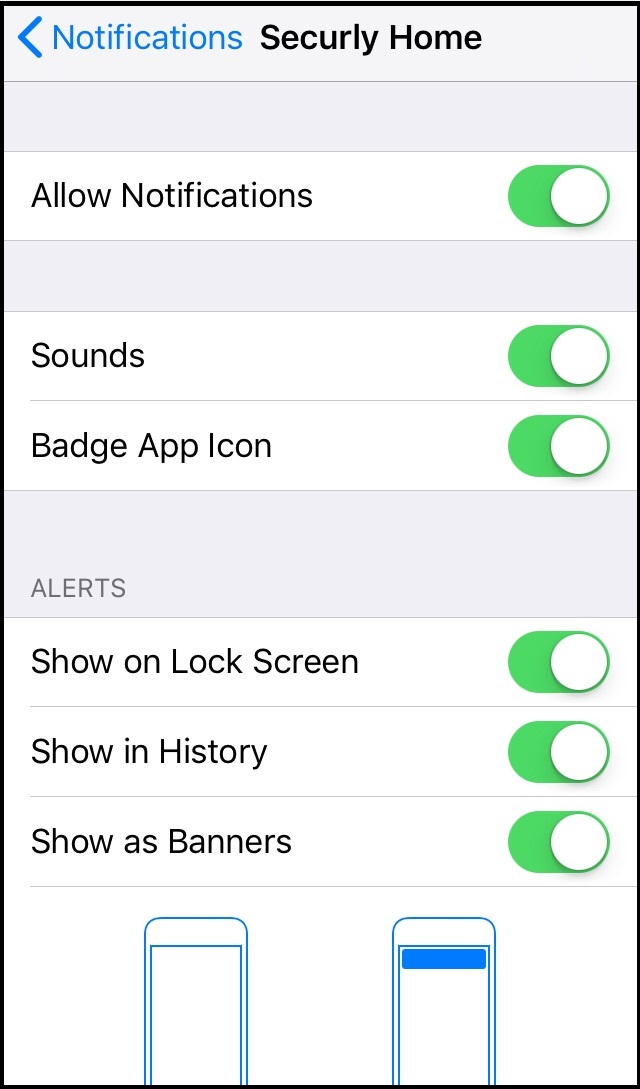In a vertically oriented rectangular interface, the top section prominently displays the word "Notifications" in blue text, accompanied by the phrase "Securely Home" in black. Below this, within a white rectangle, the text "Allow Notifications" is visible next to a green toggle switch featuring a white circle on its right side. This is followed by a light gray rectangle.

Further down, another white rectangle contains the word "Sounds," alongside another green toggle switch with a white circle on its right. Below this is the label "Badge App Icon," accompanied by a similar green toggle switch with a white circle.

This is followed by another gray section, underneath which are controls labeled "Show on Lock Screen," "Show in History," and "Show as Banners," each with identical green toggle switches and white circles.

At the very bottom of the interface, two images of cell phones are displayed side by side. The phone on the right features a blue rectangle on its screen, while the phone on the left does not have this blue rectangle.